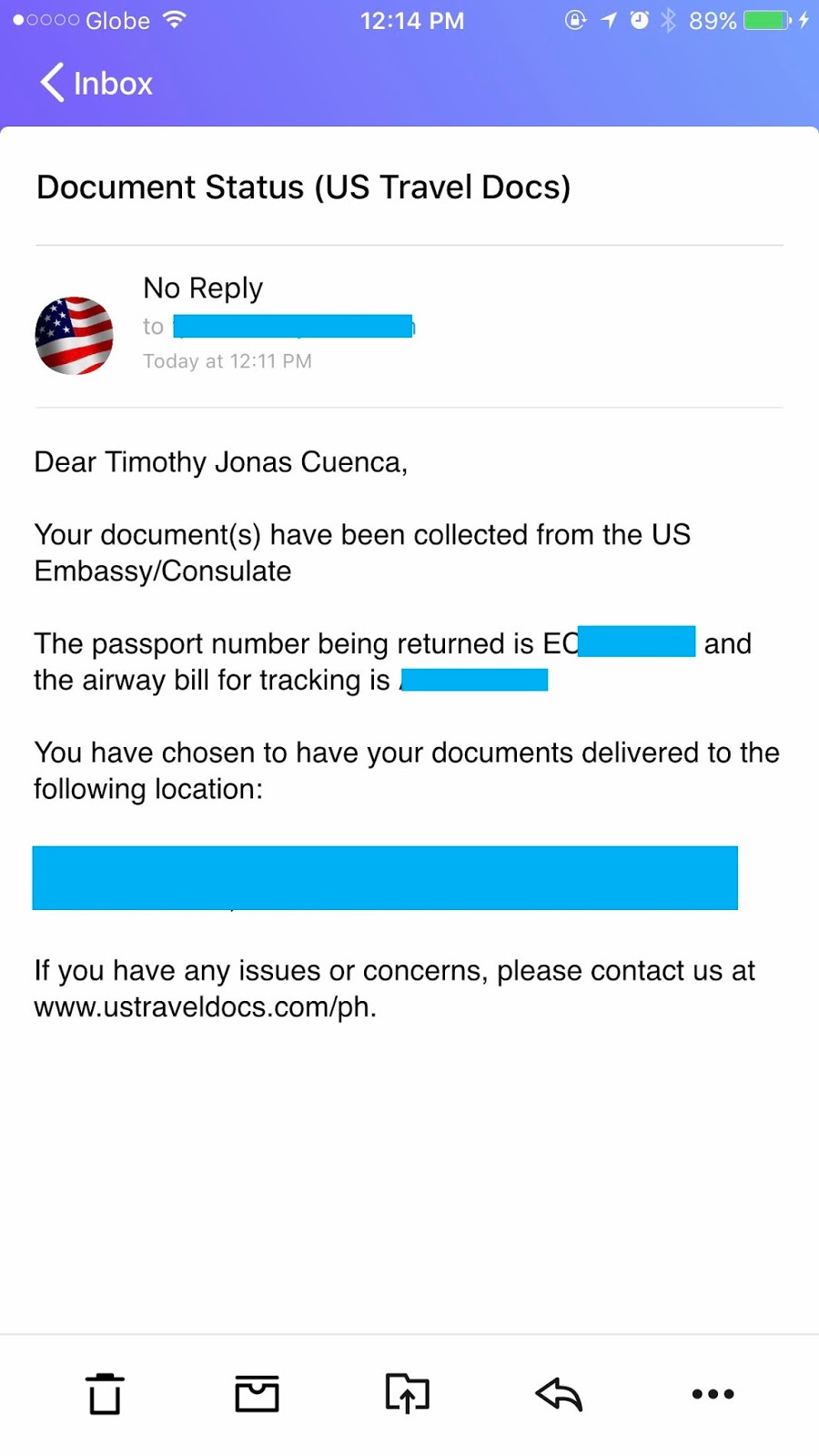A screenshot of an email viewed on a mobile device. The interface includes a top purple bar displaying phone UI elements. Beneath, on the left, is an "Inbox" label accompanied by a white back arrow. The email's subject line reads "Document Status (US Travel Docs)" and is underlined by a thin black line. Below, a section featuring a user profile picture—depicting a waving American flag—is visible. The sender's address has been censored with a light blue block. The email timestamp is marked "Today at 12:11 PM". The body of the email addresses Timothy Jonas Quinza, notifying him that his documents have been collected from the US Embassy/Consulate. It mentions the passport number, partially censored with a light blue block, beginning with "EC". Additionally, the airway bill for tracking purposes is also obscured by a blue block.